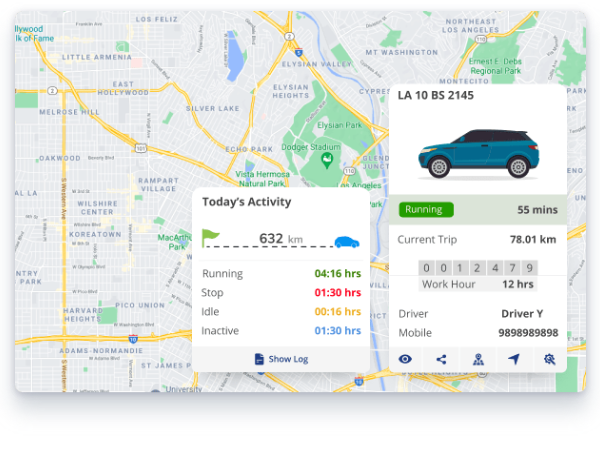In this detailed image from Google Maps, the screen displays an overview of today's activity involving a blue SUV. The vehicle has traveled a total of 632 kilometers. A green flag indicates the starting point, and a graphical representation shows the car's movement for 16 continuous hours. The statistics further reveal that the car has been idle for 6.16 hours and inactive for a substantial 130 hours. The log shows the vehicle's identifier as "LA 10 BS 2145". The current trip duration is 55 minutes, covering a distance of 78.01 kilometers. The work hours for the vehicle are recorded at 12 hours. Additional elements in the interface include icons for sharing location, settings, and navigation tools.